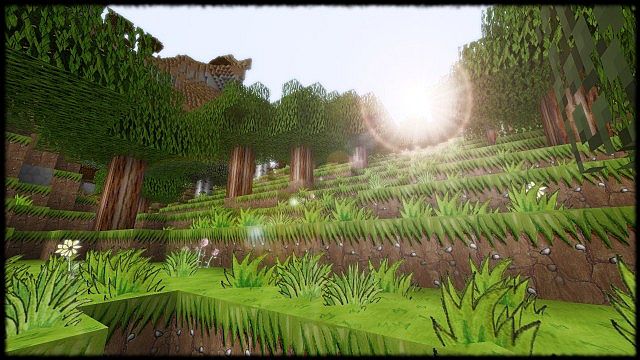A hyper-realistic or AI-generated image depicts a surreal, almost otherworldly garden scene. The garden features meticulously tiered steps adorned with vibrant, bright green grass and lush green plants interspersed with a few blooming flowers. Flanking the garden are taller trees, adding a sense of depth and enclosure to the scene. In the background, a radiant sun, encircled by a glowing white halo, rises majestically over the garden, casting an ethereal light across the landscape. This surreal illumination enhances the garden's dreamlike quality. No text or identifiable people are present in the image, although there appears to be a small, indistinct figure on the top right-hand side of one of the upper tiers. The overall effect is one of pristine beauty and serene ambiance, evoking a sense of untouched, almost fantastical nature.